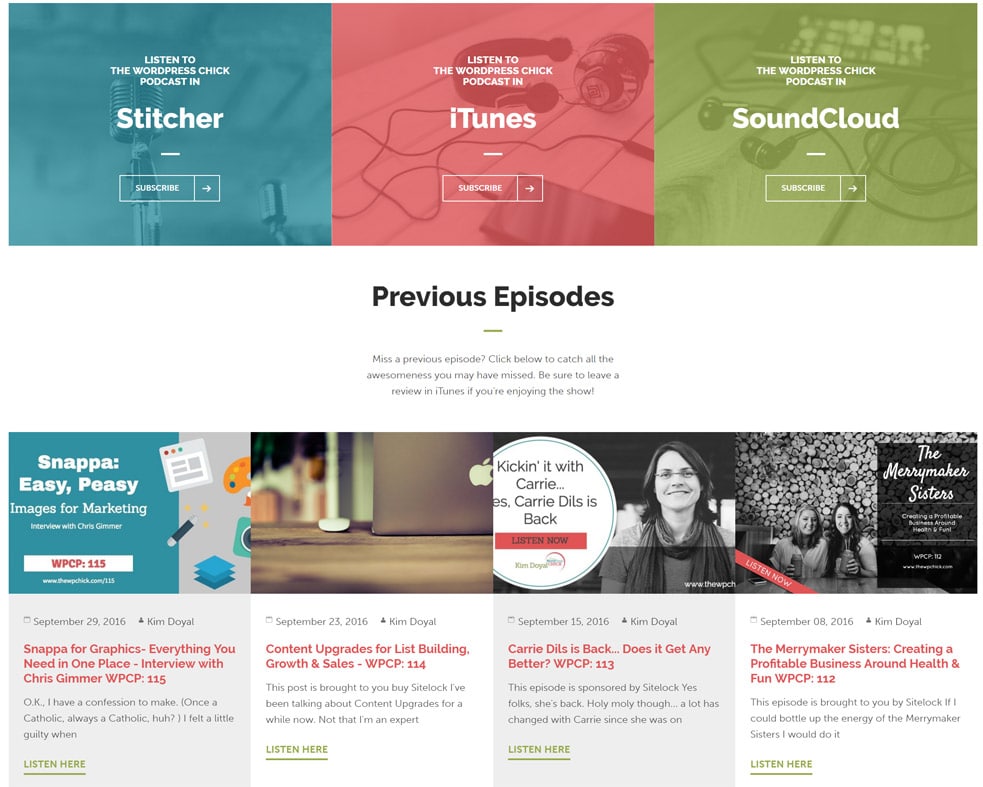The image displays a web page featuring several distinct elements. At the top of the page are three promotional banners:

1. The first banner has a light bluish tint and features an image of a microphone with a blue filter overlay. It promotes the “WordPress Check Podcast” available on Stitcher, accompanied by a "Subscribe" button and an arrow pointing to the right.

2. The middle banner sports a red filter, showcasing a pair of headphones and a phone. It advertises the “WordPress Check Podcast” on iTunes, also featuring a "Subscribe" button and an arrow pointing right.

3. The third banner is in green, depicting earbuds, and promotes the “WordPress Check Podcast” on SoundCloud. It similarly includes a "Subscribe" button along with a right-pointing arrow.

Beneath these banners, there is a section with the text: "Previous Episodes. Miss a previous episode? Click below to catch all the awesomeness you may have missed! Be sure to leave a review in iTunes if you enjoyed the show."

Following this, a series of articles are listed, each detailing different posts and their respective dates and authors:

- **September 29, 2016**: By Kim Doyle - "Snap Up Images for Marketing. Snap Up for Graphics: Everything You Need in One Place."
- **September 23, 2016**: "Interview with Chris Grammar."
- **September 23, 2016**: "Content Upgrades for List Building, Growth, and Sales."
- **September 15, 2016**: "Carrie Dills Is Back. Does It Get Any Better?"
- **September 8, 2016**: "The Merry Maker Sisters: Creating a Profitable Business Around Health and Fun."

This web page effectively integrates various promotional and informational elements to engage the visitors and encourage subscriptions and reviews.